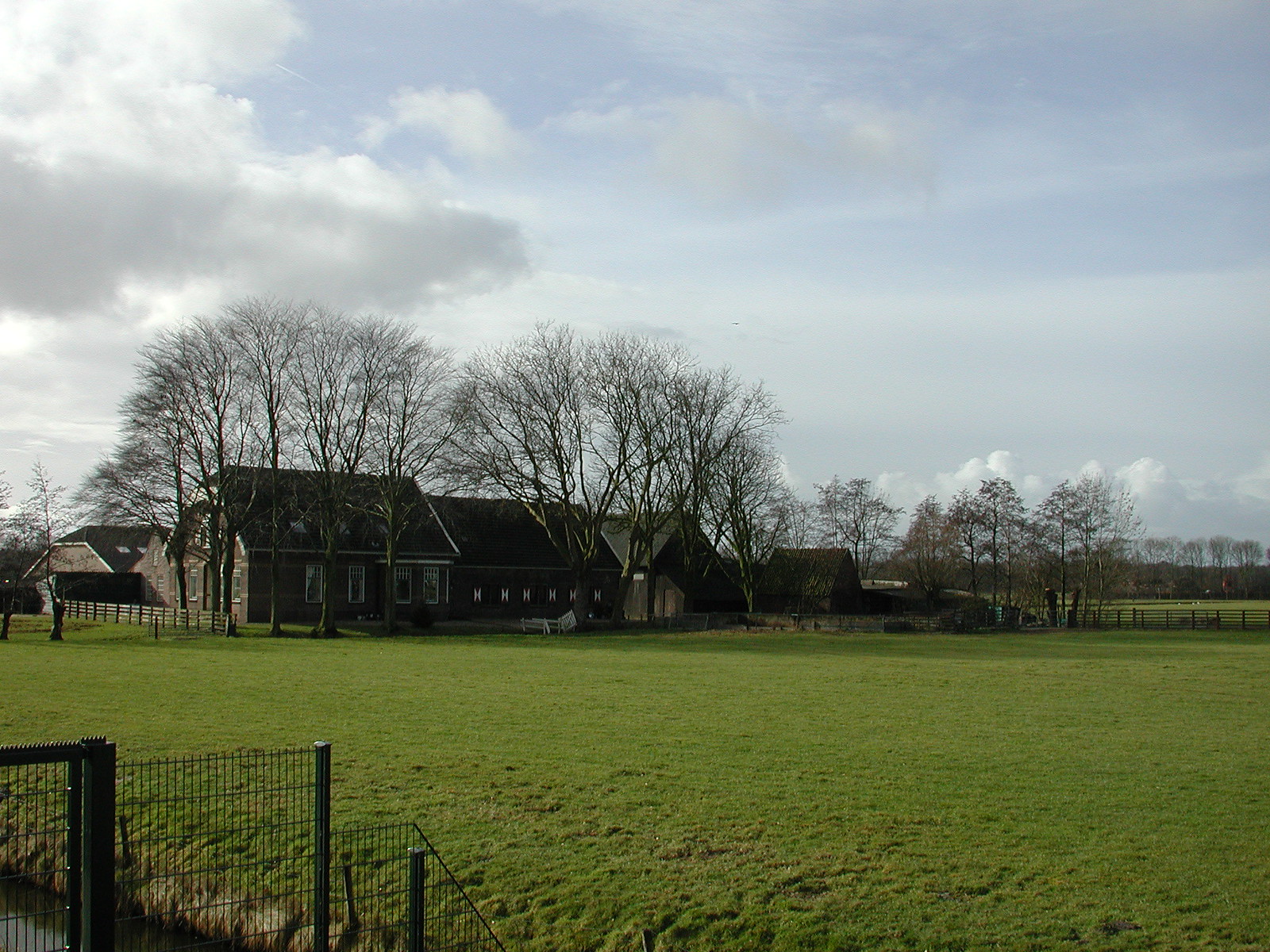The image depicts a vast pastoral farm, featuring a sizable farmhouse complex with multiple buildings, appearing to be constructed from brown brick with dark, angular roofs. The farmhouse is set amidst an expansive field of thick, yellowish-green grass, bordered by both white and metal fencing. In the foreground, the metal fencing extends towards a small stream or retention pond. Surrounding the farm are numerous trees, all barren of leaves, suggesting the season might be late fall or early spring. The sky above is a mix of hazy light blue and various gray clouds, providing a peaceful yet overcast atmosphere. The overall setting reflects a serene and private property with significant acreage, characterized by its classical architectural elements and the calm, natural landscape.